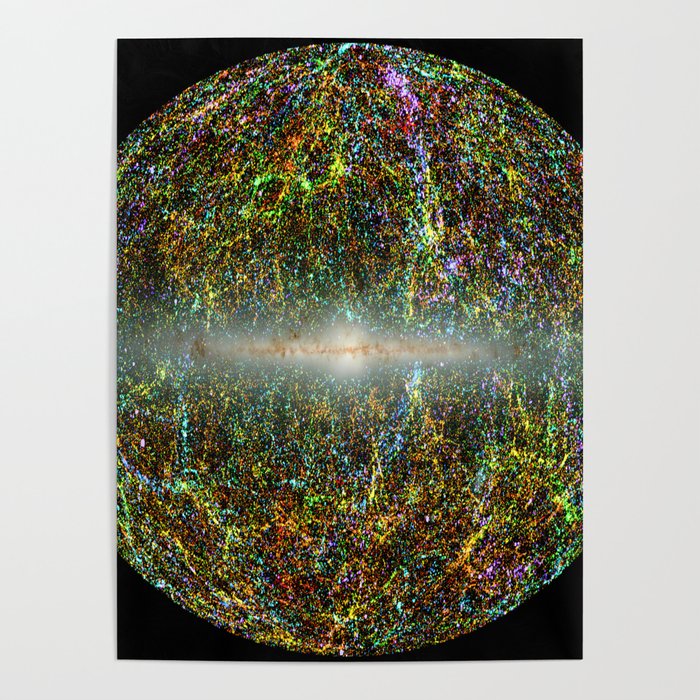The image showcases a vibrant abstract art piece set against a light gray wall, digitally edited to simulate it being displayed in a living space. The art itself features a black background with an eclectic sphere of random neon colors including yellows, greens, oranges, blues, purples, and pinks, radiating in no particular pattern. At the center of this colorful sphere, a white, cloudy blur horizontally spans across, accentuated by brown squiggle marks that seem to dance from right to left. This visually striking poster captures the viewer's attention with its chaotic yet mesmerizing display of colors.